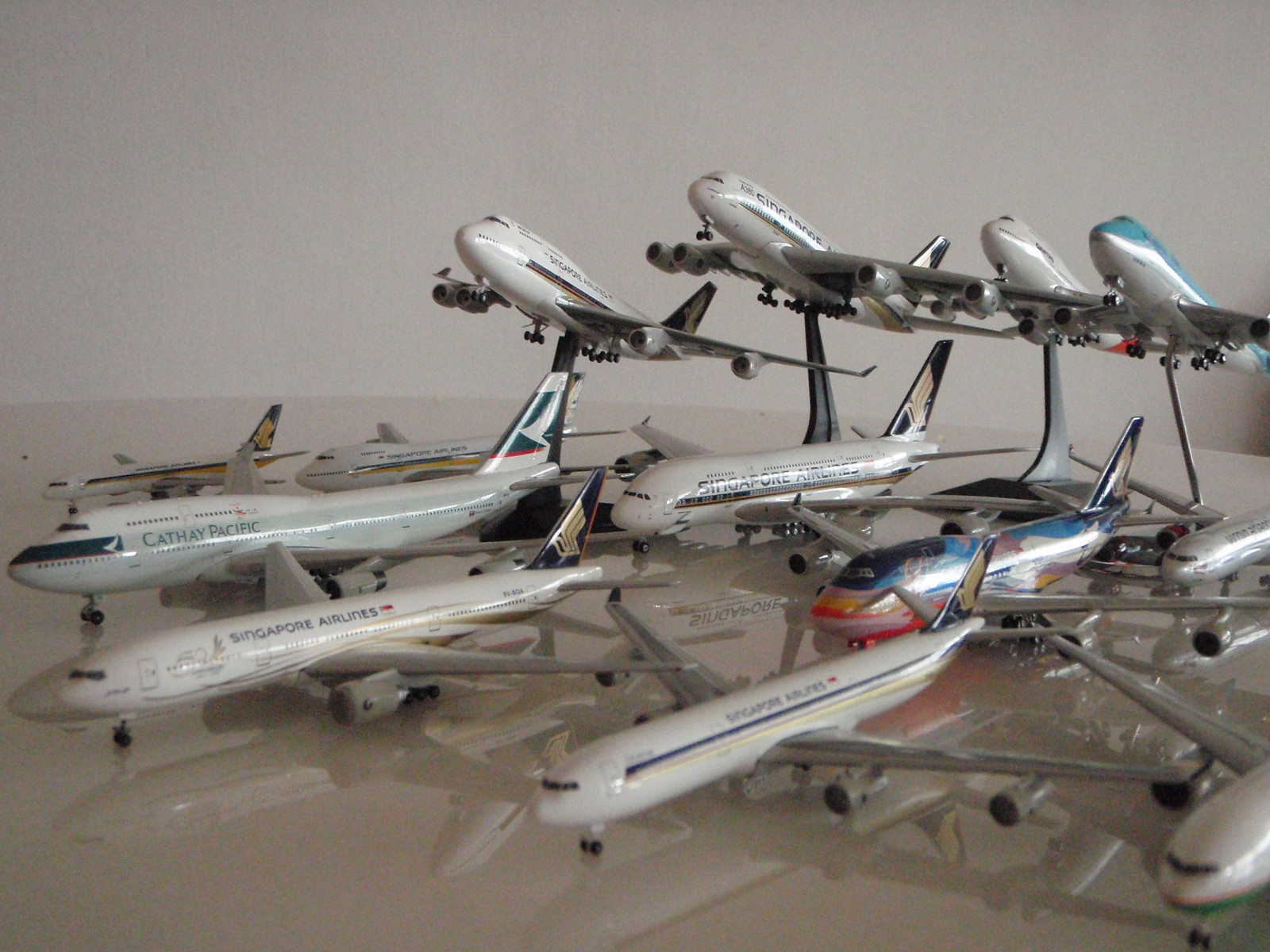The image features a round, opaque glass table with a mirror-like reflective surface set in a white room where the wall behind appears to be a light grayish beige. Displayed on the table are approximately 13 or 14 meticulously detailed model airplanes. Among them, several models represent Singapore Airlines, distinguished by various designs including one with a black tail and gold accents, and another with blue and yellow stripes. One prominent model aircraft is a jumbo jet labeled Cathay Pacific, characterized by its red, white, and blue front and similarly colored tail fin. A striking, colorful plane that seems to have a graffiti-like design adds a vibrant touch to the otherwise polished collection. The planes reflect off the table's shiny surface, creating an illusion of them being suspended mid-air, poised for takeoff. Some models are seen elevated, possibly balanced by string, enhancing the dynamic lifelike presentation of this commercial airplane collection.